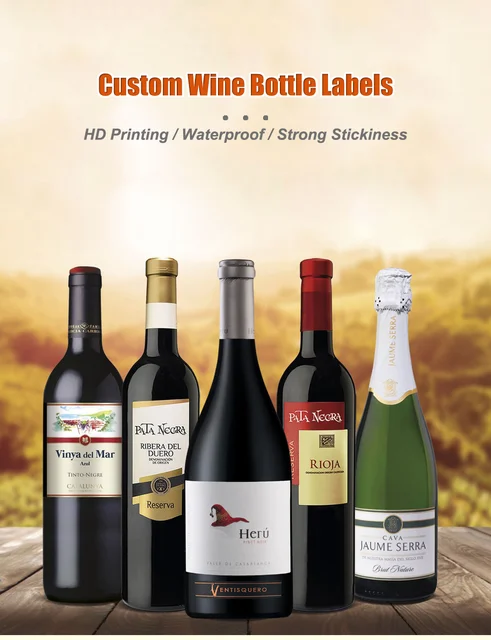The image showcases five wine bottles meticulously arranged on what appears to be a picnic table, with only a portion of the table visible at the bottom edge of the photo. The upper part of the image features a gradient background transitioning from a light tan to white, decorated with text in a distinctive red font that reads: "Custom Wine Bottle Labels...". Below this, a description highlights, "HD Printing / Waterproof / Strong Stickiness," emphasizing the quality of the labels.

Behind the bottles, the backdrop displays a picturesque scene resembling a yellowish-bronze field or a sunlit mountaintop, contributing to the image’s warm and inviting atmosphere. The wine bottles themselves are predominantly black, lending an air of sophistication, with the exception of the far-right bottle, which stands out due to its green hue. This contrast adds visual interest and variety to the composition, making each bottle uniquely appealing.